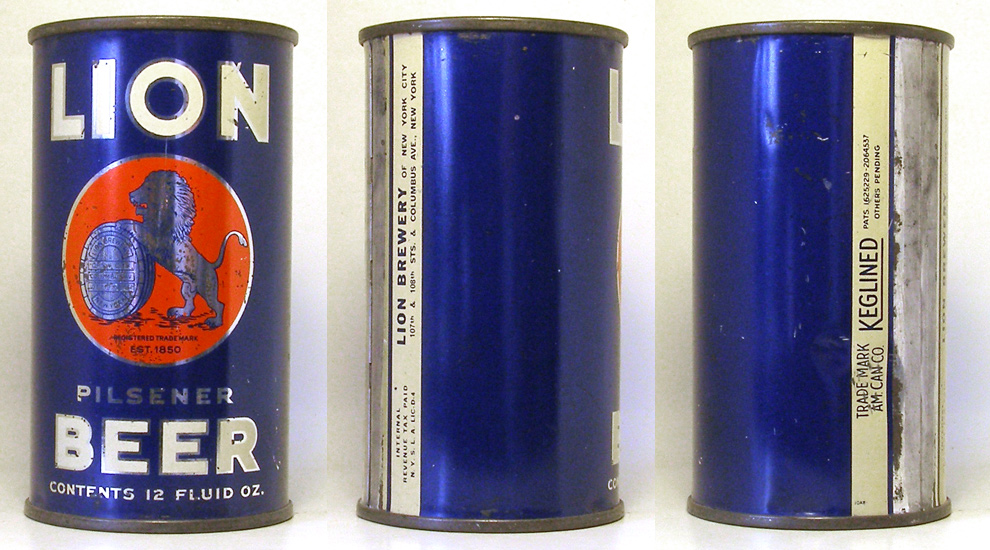The image depicts an ad featuring three beer cans, all displaying different angles of Lion Beer cans. The cans are a rich, dark blue color, with bold white uppercase letters spelling out "LION BEER" on the front of the leftmost can. Between "Lion" and "Beer" is a distinctive emblem: a silver circle with a red interior, showcasing a lion upright on its hind legs, with its front paws resting on what appears to be a large coin. Below this emblem, in smaller white letters, the word "PILSNER" is visible, followed by "CONTENTS 12 FLUID OUNCES" at the very bottom.

The middle can is partially facing the viewer, revealing the text "LION BREWERY" on a white vertical banner, which continues with "NEW YORK CITY" and an obscured address on Columbus Avenue.

The rightmost can displays the text "KEG LINED", emphasized with an underline. The can also mentions "TRADEMARK AM CAN CO." along with some unreadable smaller text. Each can features a silver rim at the top and bottom, adding to the overall sleek metallic aesthetic. This trio of cans, set against the blue background, collectively highlights the brand's striking design and signature details.